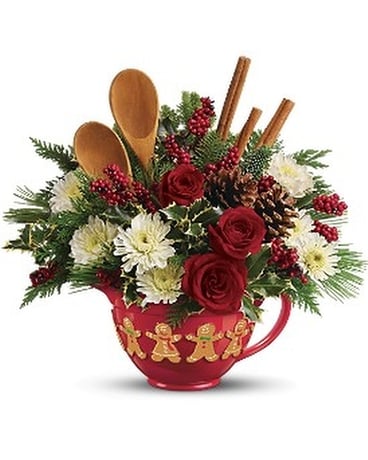This digital photograph, set against a completely white background, showcases a festive, holiday-themed red container, which could be described as a vase, pot, or even a watering can. The container features a right-sided handle and is adorned with four spaced-out gingerbread men in brown, white, red, and green colors. The container holds an elaborate, colorful bouquet. Visible within the arrangement are striking red roses, white flowers with yellow centers (resembling daisies), green pine needles, and red berry-like details that evoke cranberries. Adding to the festive theme, the bouquet includes brown pine cones on the left side, three cinnamon sticks on the right, and two lightly tanned wooden kitchen spoons.